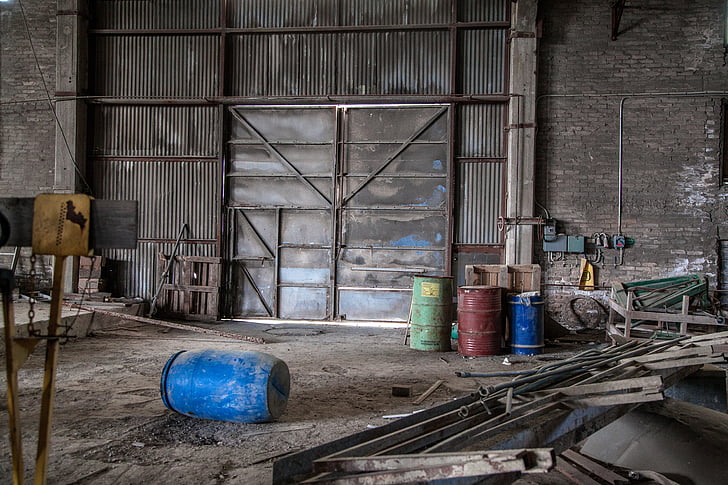The image depicts a partial view of an industrial building's interior, possibly an abandoned warehouse. The backdrop features two closed metal double doors surrounded by corrugated metal sheets arranged vertically. The right wall is composed of dirty brown bricks, interspersed with blue electrical boxes and a conspicuous red button connected to several pipes. In the foreground, scattered pieces of rusted metal beams and pipes litter a rocky, dirt-like floor. A blue plastic barrel lies on its side to the left, adjacent to a sign on a wooden post with black ends forming a T-shape. Nearby, a tipped-over blue wheelbarrow and additional barrels in red, green, and blue colors are visible, along with a wooden crate. The upper left corner of the image shows wires hanging down from the ceiling. The overall color scheme of the image is predominantly gray, reflecting the industrial and aged nature of the setting.